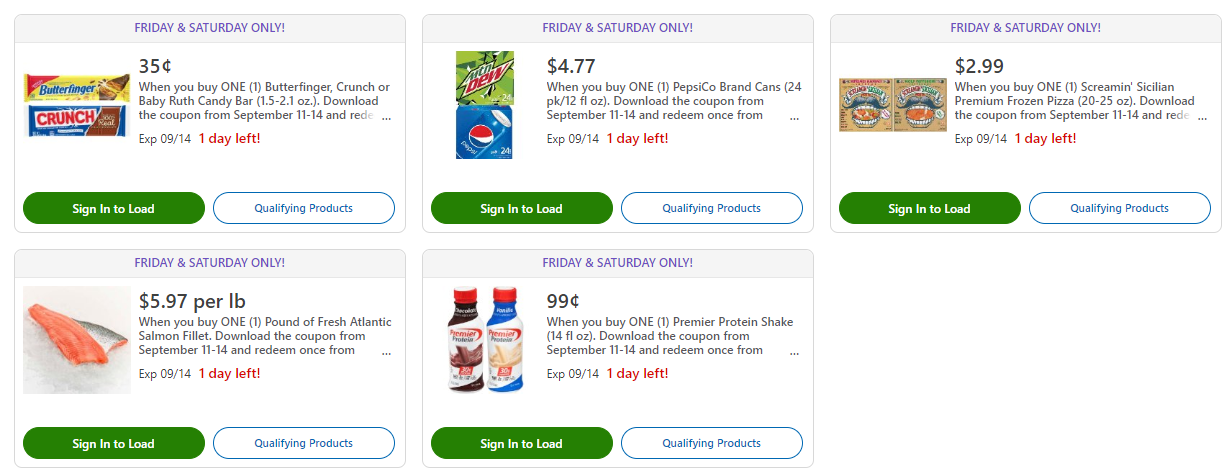The screenshot depicts a section of a web page arranged in a three-column, two-row format, featuring a total of five cards. Each card is meticulously designed to advertise a product and consists of several distinct elements:

1. **Header:** The header of each card prominently displays the text "Friday and Saturday Only," possibly indicating a limited-time promotional offer. Additionally, it includes an expiration date and the number of days left in the promotion, all in a bold font to catch the viewer's eye.

2. **Image and Text Layout:** Within the body of each card, there is an image positioned on the left side, showcasing the product in question. To the right of the image, there is a section of text that resembles a short paragraph, detailing specific features and benefits of the product. The text is likely concise and informative, aimed at enticing potential buyers.

3. **Buttons:** At the bottom of each card, there are two call-to-action buttons. The left button is a rounded rectangle with white text on a green background, about half the width of the card, and is labeled "Sign In to Load." The right button features blue text on a white background with a blue border and is labeled "Qualifying Products."

Each card is designed with ample padding and margin, ensuring a clean, visually appealing layout. Prices are bolded within the text to immediately draw attention, reinforcing the promotional aspects of the offers being highlighted.